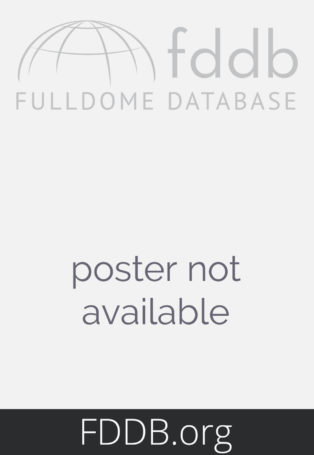The image predominantly features text against a white background. At the top, there is a light gray, dome-shaped logo, resembling the wireframe top of a birdcage, without the bottom portion. To the right of the logo are the letters "FDDB" in gray, followed by the full name "FULL DOME DATABASE" in all capital letters below it. The majority of the image consists of white space. About two-thirds down, centered in dark gray lowercase text, are the words "poster not available." At the very bottom, a black rectangular stripe spans the width of the image, containing the text "FDDB.org," with "FDDB" in uppercase and "org" in lowercase, in white letters.